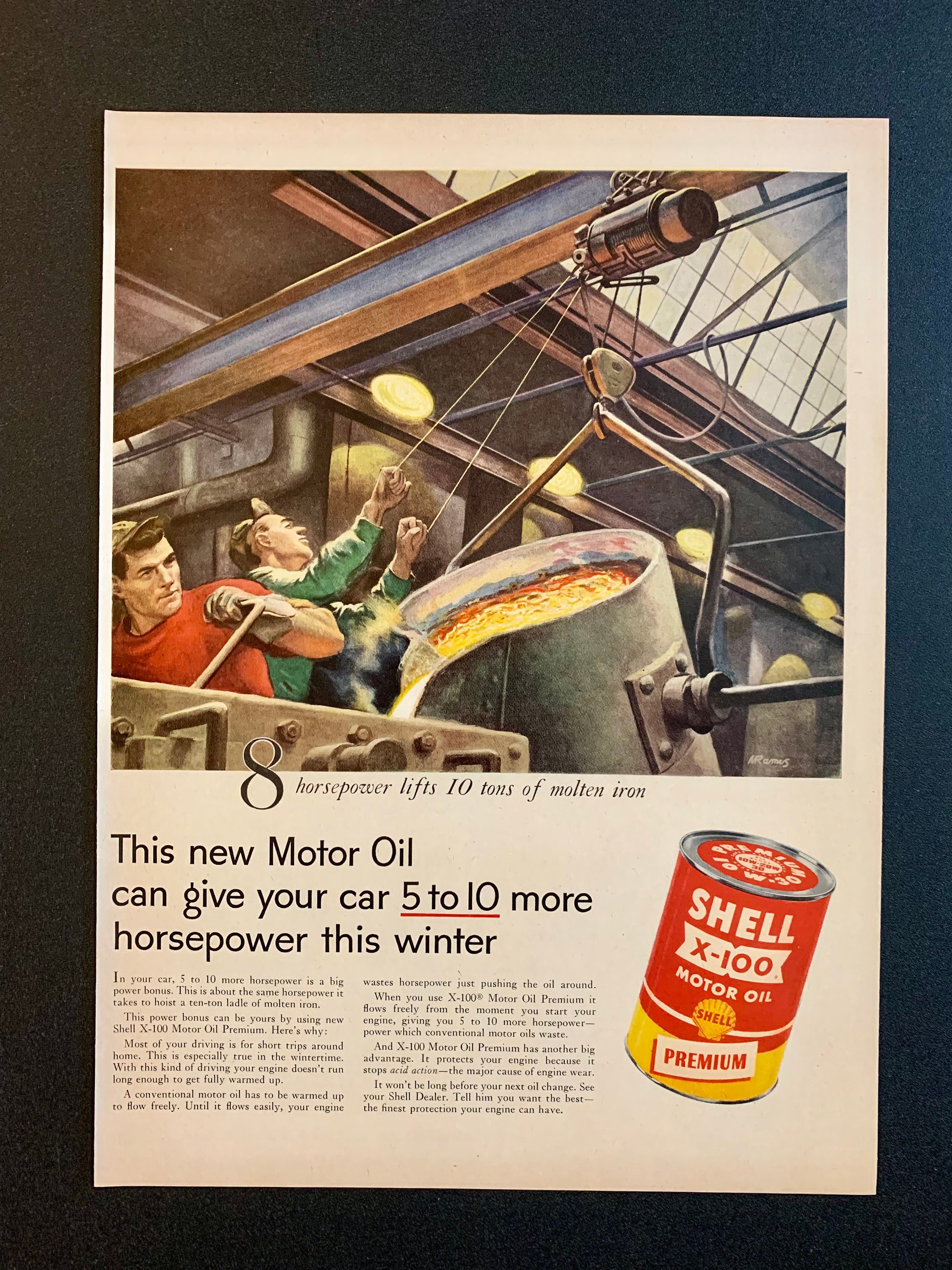The image resembles an old magazine advertisement with a predominantly black background that fades into a darker tone at the lower left corner and brightens up to a bluish hue on the upper right and left. The main visual attraction is a square illustration at the top, portraying a steel mill scene where two iron workers are seen manipulating a large pot of molten iron. The worker on the left, wearing a red shirt, appears to be controlling the operation, while the one on the right, dressed in a green shirt, is pulling a string to pour the molten iron. A caption beneath this illustration boldly states in black text: "8 horsepower lifts 10 tons of molten iron."

On the lower right of the advertisement, there is a vivid photo of a can of Shell X-100 motor oil. The can features a red and yellow label with the recognizable Shell logo and the word “Premium.” Adjacent to it, on the left side of the image, substantial black text highlights the benefits of this new motor oil, claiming it can provide your car with an additional 5 to 10 horsepower this winter. Two detailed paragraphs below the main message further elaborate on the capabilities of the motor oil. This blend of illustration and photography against the contrasting black background creates a striking and memorable advertisement.